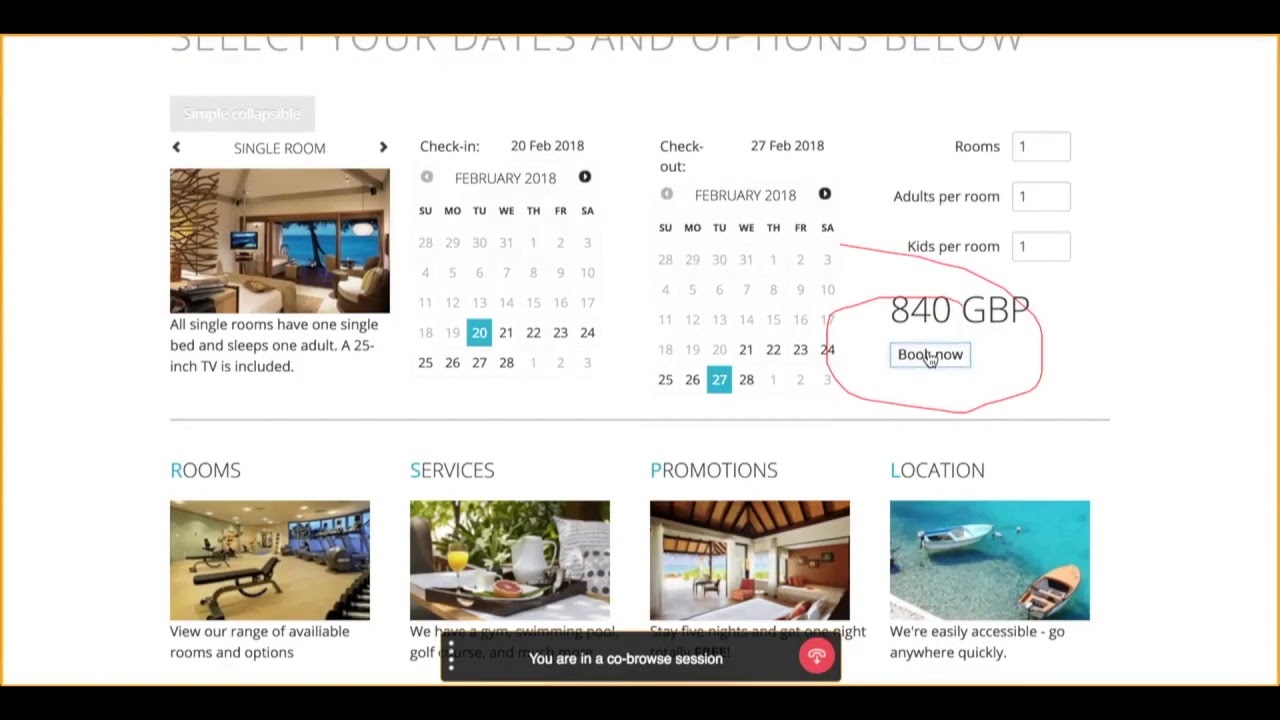A screenshot with a white background, featuring detailed information about a room booking. The screenshot encompasses a lecture date, a calendar, and various booking options. Below the information, there is an image of a single room, which contains one single bed and accommodates one adult. Included in the room is a 25-inch TV. The calendar displayed is for February 2018, and specific dates are highlighted: check-in is marked with a blue square behind February 20, 2018, and check-out is similarly marked behind February 27, 2018. 

The booking details reveal one adult per room, with an additional allowance for one child. The total cost of the stay is 840 GBP, highlighted with a red line, alongside a "Book Now" button. Additionally, the screenshot provides options to view a range of available rooms, details on the property's convenient location, and information about related services and ongoing promotions.